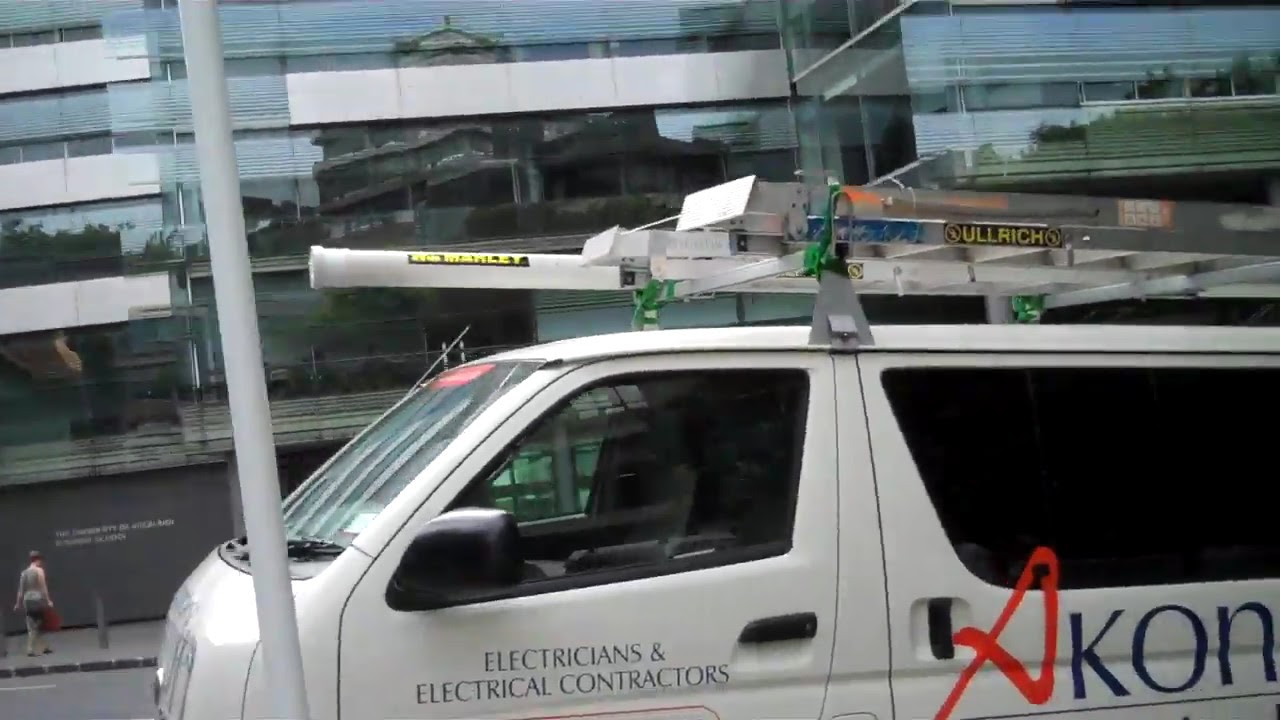The image depicts a white electrician's van parked on a city street, prominently framed against a backdrop of modern, metallic-glass buildings at least three stories high. The van's design and markings suggest it belongs to an electrical contracting company, with "electricians and electrical contractors" written in blue on the driver's door. The van features semi-tinted front windows and fully tinted back windows. A red sideways triangle and the letters "KON" are visible on the sliding door, possibly indicating the company name. Positioned on the roof rack are multiple ladders and cylindrical tools, further emphasizing its work-related purpose. In the foreground, near the front of the van, stands a street pole, while the sidewalk below stretches into the distance where a woman is seen standing, her arms by her side. Reflections of surrounding buildings are mirrored in the skyscraper's glass, reinforcing the urban setting of the scene.